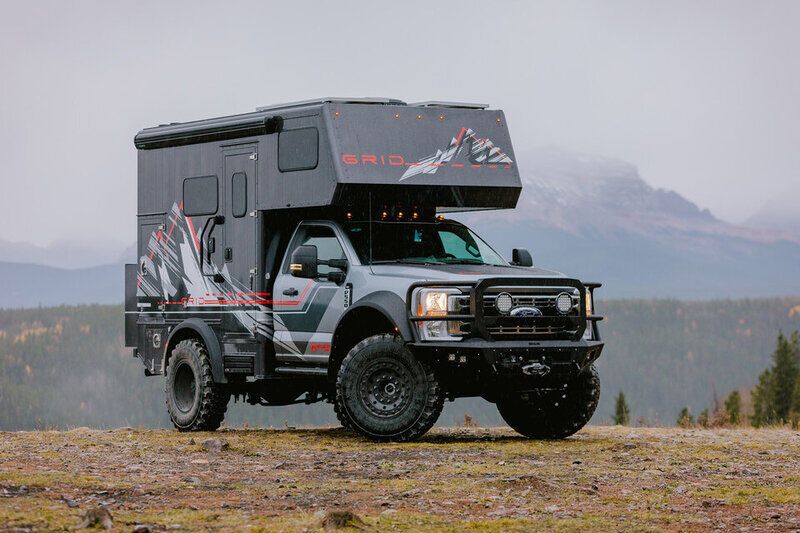The image depicts a rugged, black (or possibly gray) Ford pickup truck outfitted with a camper shell, parked on a ridge in a mountainous recreation area. The truck, which has tinted windows and an extra bar across the grill for pushing, features a distinctive decal that extends from the side door to the cab, showcasing a design that includes red, black, white, and gray tones, reminiscent of a mountain range. The word "GRID" is prominently displayed on the camper shell near the top, with a logo to the right of it. The backdrop includes a rugged dirt area with sparse grassy patches and rocks, surrounded by layers of evergreen trees, extending to imposing, overcast mountains in the distance. The sky above is a mix of gray clouds and patches of blue, contributing to an overall foggy and overcast ambiance.